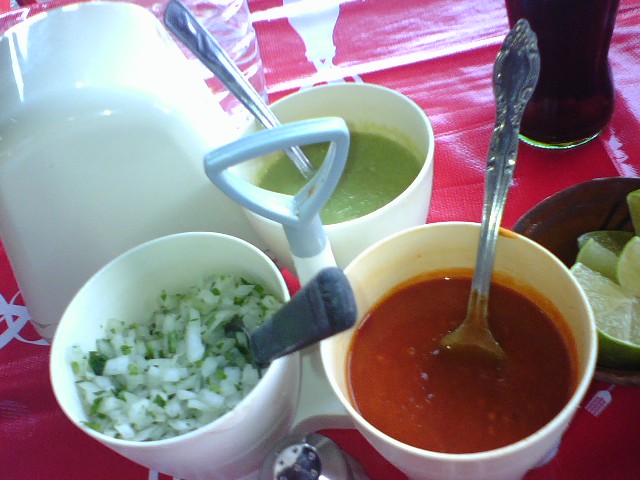In this vibrant photograph taken from a slightly top-down angle, a trio of sauces sits prominently on a red tablecloth, which hints at a lively restaurant setting. The three tall, white plastic cups in the foreground contain flavorful toppings for dishes, possibly for tacos given the context. The leftmost cup brims with finely chopped onions, complemented by what appears to be green onions or cilantro, with a black plastic spoon protruding from it. Directly behind it sits a textured light-green sauce, likely guacamole, in which a silver spoon is lodged. The rightmost cup holds a bright red salsa, also with a silver spoon dipping into it. Adjacent to these, a small dark brown plate contains freshly sliced limes, their juicy interiors clearly visible. In the top right corner, a glass bottle of Coca-Cola, resting against the red polyester nylon tablecloth, adds a classic touch to this rich and colorful scene reflective of a bustling Mexican restaurant.